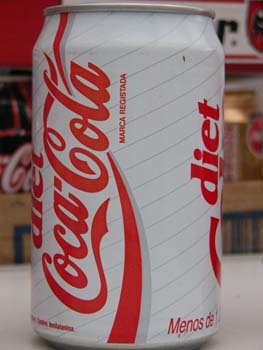The image prominently features a close-up of a Diet Coca-Cola can set on a white counter. The can itself is distinctive with a white background adorned with gray diagonal stripes spiraling around it. The iconic Coca-Cola script in bold red lettering spans diagonally across the can, with the word "Diet" partially visible at the top and extending towards the left of the can. Below this, in red text, is a foreign phrase starting with "M-E-N-O-S D-E," alongside "Marca Registrada" indicating it might be a vintage or international design.

The can’s edges are silver and rounded, giving it a vintage feel. In the blurred background, additional Coca-Cola logos are visible, with various colors and another partial "C" of a logo discernible. The background gives an impression of being in a store or food court with more cans and Coca-Cola branding subtly peeking through from behind. The overall framing of the image is vertical, emphasizing the sleek and classic design of the can against the minimalist white surface.